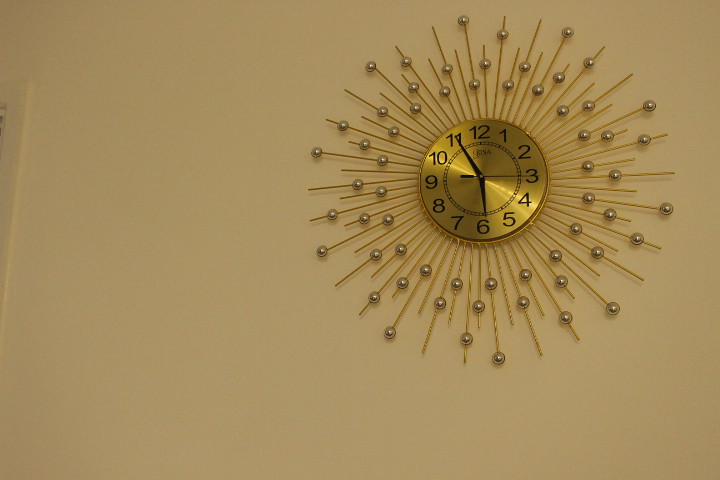This photograph features an ornate golden clock mounted on a wall with a golden brown or beige hue. The clock's face is gold-colored, displaying plain black numbering from 1 through 12. Black hands indicate the time as 5:55. Surrounding the clock face, a smaller inner circle features intricate black designs. Extending from the clock are numerous golden rods of varying lengths, each adorned with one or two silver beads, creating a starburst or sunburst effect. This decorative motif gives the clock a striking, radiant appearance. The clock is positioned in the upper right-hand corner of the image, and a slight glimpse of a doorframe from an adjacent room is barely visible.